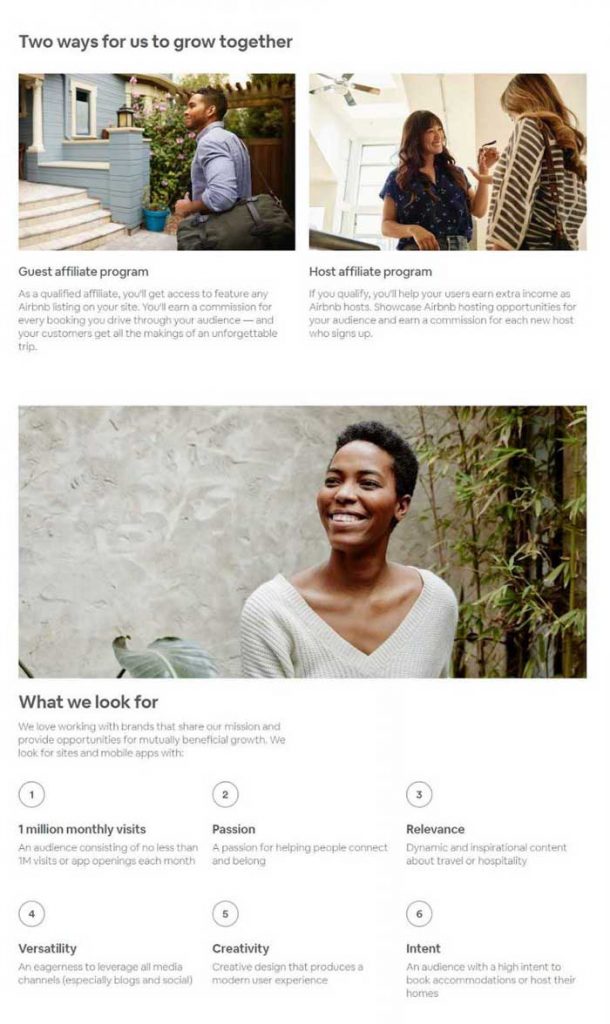**Descriptive Caption for Image:**

The page presents two distinct pathways for collaboration labeled under "Two Ways for Us to Grow Together." The first section, titled "Guest Affiliate Program," features an image of a Black man donning a blue shirt, carrying a brown or grayish duffel bag under his arm as he walks towards a house. The house is light blue with white trim and features a lantern by the entrance. Its four concrete, whitish-colored steps lead up to the door, enhancing the welcoming ambiance.

Adjacent to it is the "Host Affiliate Program," exemplified by an image of two women engaging in conversation inside a home. The interior is characterized by a palette of white and off-white tones, complemented by a darker-colored ceiling fan. The woman on the left sports long dark hair and a dark shirt, while the woman on the right has blondish hair and wears a striped shirt, depicting a scene of warm, in-house interaction.

Further down, the section titled "What We Look For" showcases a cheerful Black woman standing outdoors beside a potted plant. She is wearing a white sweater and gazes upwards with a smile, encapsulating the positive spirit desired in affiliates. Below her image, the criteria for selection are listed, including:

1. One Million Monthly Visits
2. Passion
3. Relevance
4. Versatility
5. Creativity
6. Intent

Each bullet point is followed by detailed descriptions, highlighting the qualities and expectations from potential affiliates.